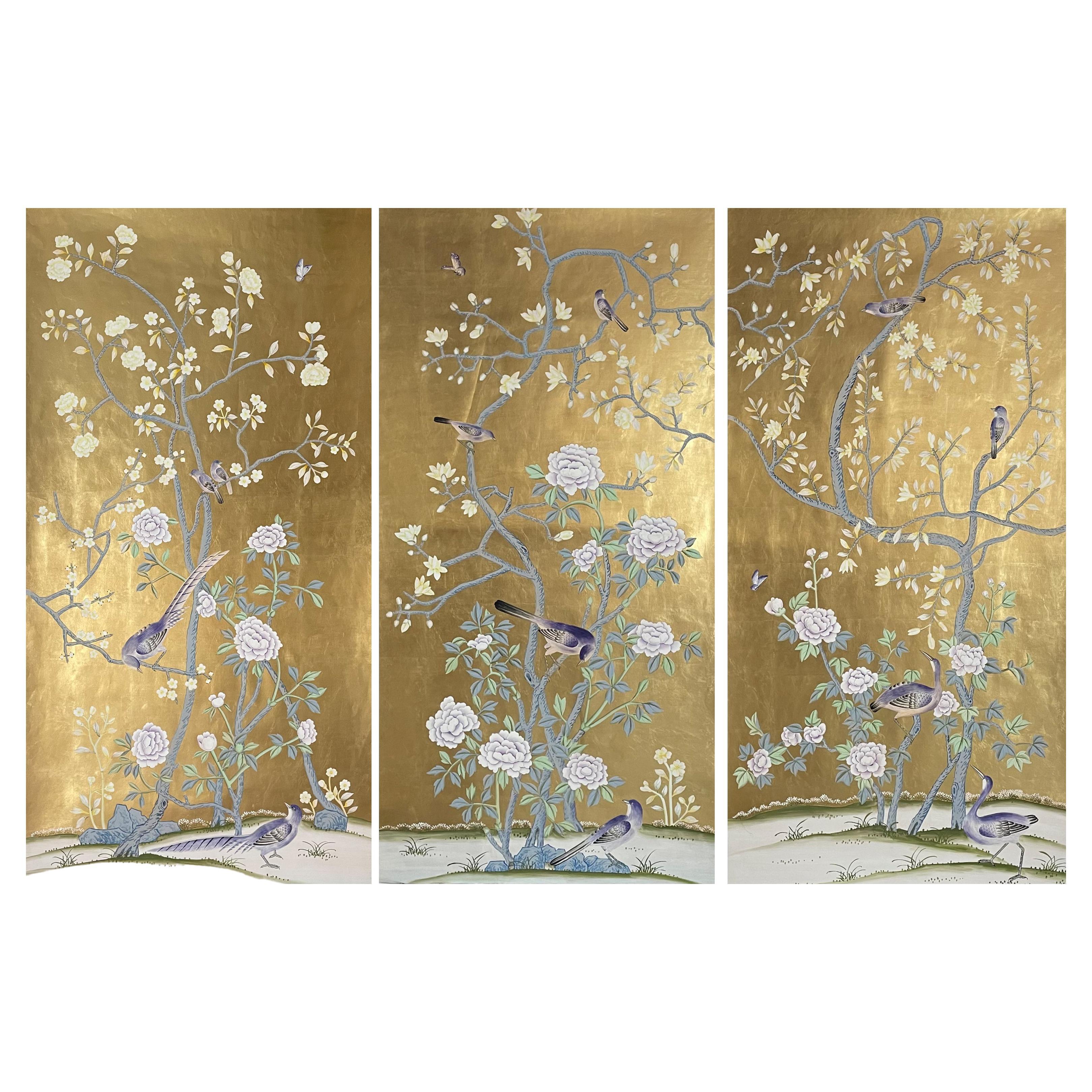This artwork consists of three equal-sized panels that form a cohesive, side-by-side triptych. Each panel features a consistent golden, shiny background with a white ground surface, resembling either sand or snow, indicative of a winter scene. The primary focal points in all three panels are intricately depicted gnarly trees adorned with light purple and light yellow flowers. These trees host a variety of gray birds, some perched on the branches and some wandering on the ground, contributing to the liveliness of the scene. 

In the left panel, two large birds with long tails and two smaller birds occupy different heights on the tree. In the central panel, the bird on the ground is positioned looking upward at the larger bird in the tree, while the two smaller birds are now spaced further apart in the upper part of the tree. Finally, the right panel presents a bird on the ground with a notably long neck, mirrored by another long-necked bird perched in the tree, both looking upward; two small birds remain higher up in the tree.

Each panel is triangular and showcases delicate bushes or small trees with sparse leaves, enhancing the artwork's delicate and intricate nature. The positioning of the birds varies among the panels, creating a dynamic and interconnected scene that may evoke a Japanese aesthetic. All panels together highlight harmonious elements with slight variations, enriching the visual narrative across the triptych.